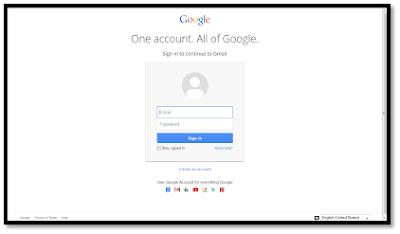The image displays a Google account sign-in page, framed within a black square, resembling a screenshot taken from a computer screen. The background of the page is predominantly white. At the very top, centered, lies the Google logo featuring the blue capital 'G', red lowercase 'o', yellow lowercase 'o', blue lowercase 'g', green lowercase 'l', and red lowercase 'e'. Below the logo, in a dark gray color, the text reads, "One account. All of Google." 

Beneath that, there is a smaller, hard-to-read message in the same dark gray color that likely states, "Sign in to continue to Gmail." 

The central part of the page features a light gray-shaded square with a placeholder for a user's profile picture or avatar at the top. Directly below this, there is a white rectangle outlined in blue, labeled "Email," where users would input their email address. Beneath the email field is another white rectangle labeled "Password," intended for password input. At the bottom of this section, a blue button with white text reads "Sign in." 

Additionally, there is a faintly visible option below the sign-in button, which appears to be a checkbox for staying signed in, though the text next to it is not clearly legible.